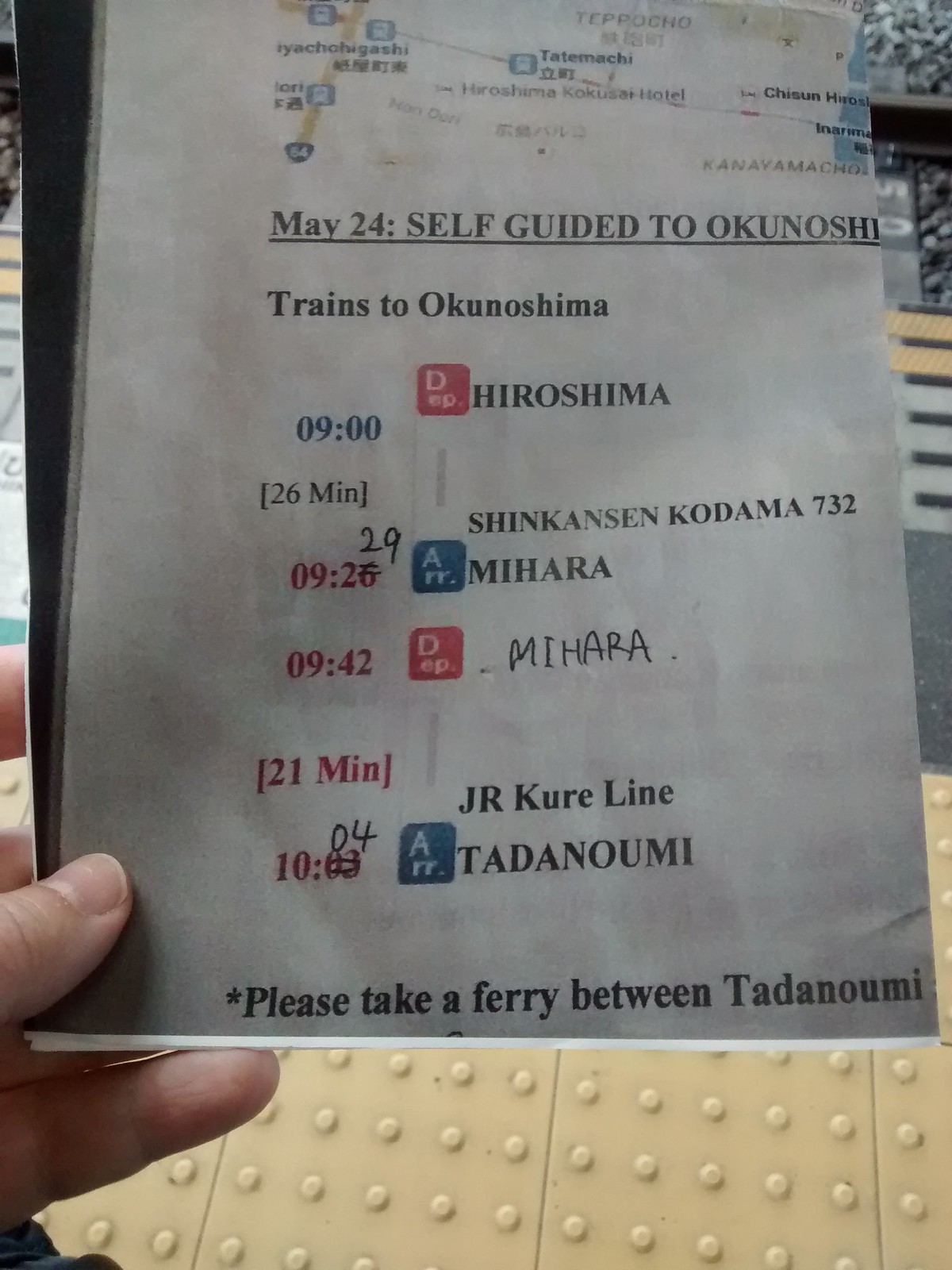The image depicts a printed photograph of a travel itinerary held by a person's hand with visible fingers on the left side. The setting is on the edge of a train platform characterized by yellow textured tiles with raised dots, designed to prevent slipping, with train tracks and gravel visible below. The itinerary on the paper marks May 24 with a self-guided tour to Okunoshi, underlined in the center in black print. Below this headline, it details various train schedules starting from Hiroshima at 9:00 AM, where a note indicates a correction in the travel time from initially written 26 minutes to 29 minutes via Shinkansen Kodama 732. The subsequent stop is Mihara at 9:42 AM, with another correction changing 10:03 to 10:04 AM, covering a 21-minute journey via JR Kure Line to Tadanoumi. There are also colorful markers - a red square next to Hiroshima, a blue square next to Mihara, and another blue square for Tadanoumi. An important note at the bottom, partially obscured by fingers, advises taking a ferry between Tadanoumi and another location. The background features a map with Japanese place names and train station symbols, although specifics are cut off due to the angle and the cropping of the image.